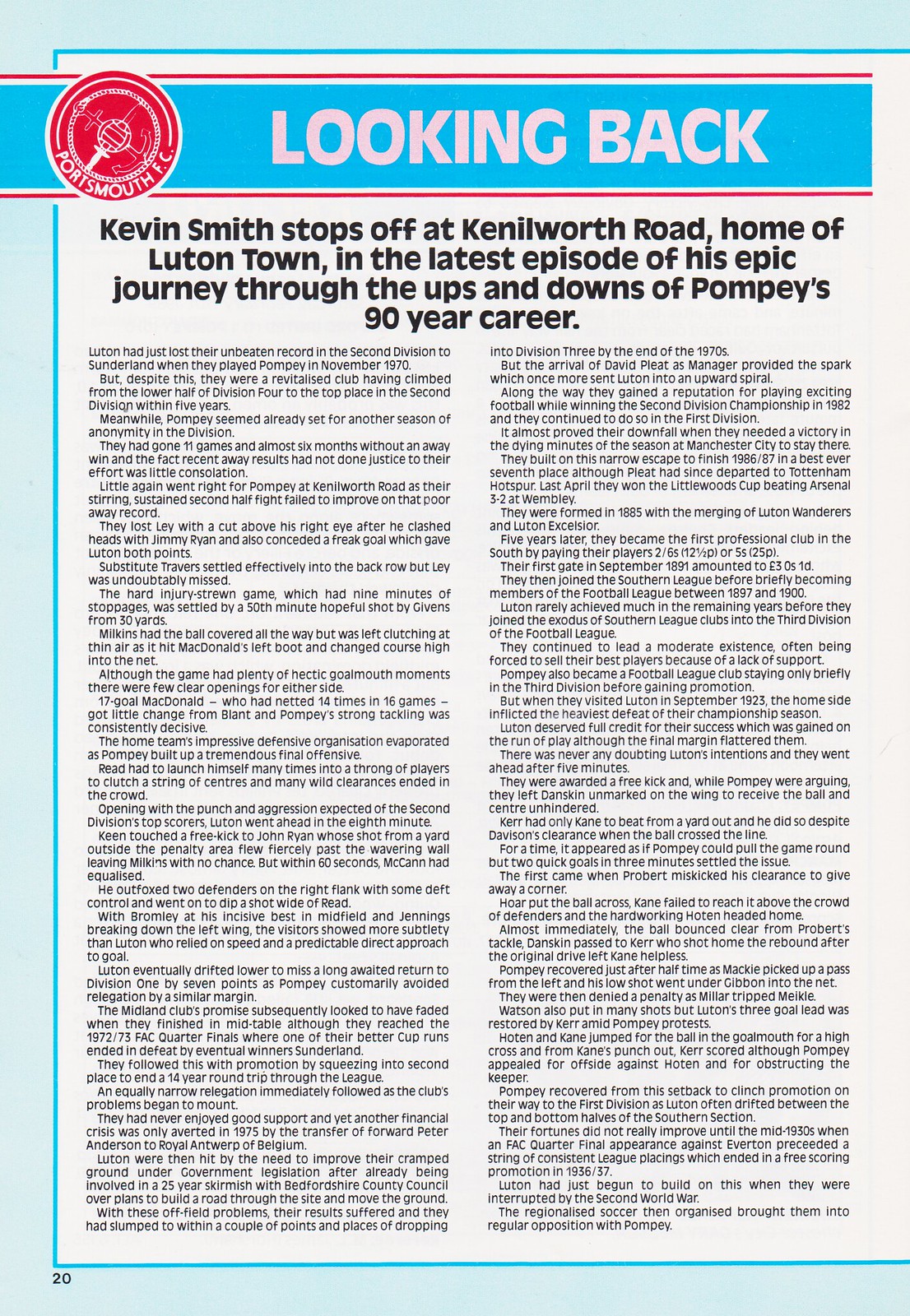This flyer features a clean, white background with a distinct blue border along the top, left, and bottom edges. At the top, a baby blue banner prominently displays the title "Looking Back" in pink lettering. Adjacent to the title is a red, circular insignia with a soccer ball in the center, labeled "Portsmouth FC," indicating its association with the Portsmouth Football Club. Below the title, in black lettering, is a headline that reads, "Kevin Smith Stops Off at Kenilworth Road, Home of Luton Town, in the Latest Episode of His Epic Journey Through the Ups and Downs of Pompeii's 90-Year Career." The rest of the flyer is densely packed with small, cramped text detailing Kevin Smith's career highlights, challenges, and significant events. The article appears lengthy, attempting to condense a substantial amount of information onto a single page, making it rich in detail and narrative.